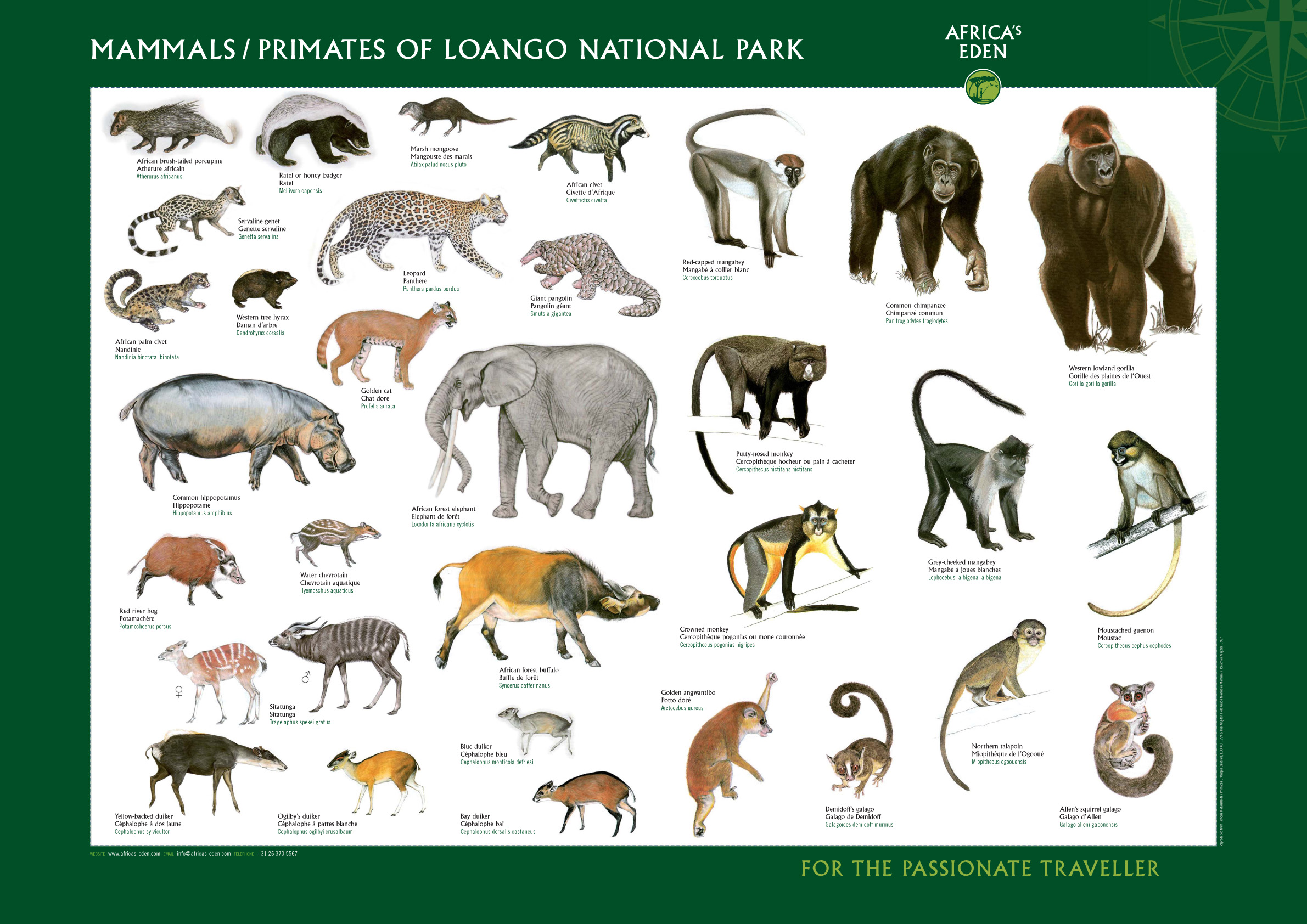This detailed infographic showcases a diverse array of mammals and primates found in Luongo National Park, set against a crisp white background framed by a green border. In the top left corner, white text labels the image as "Mammals/Primates of Luongo National Park," while to the right, the title "Africa's Eden" is accompanied by a green circle within the border. Notable animals featured include gorillas, different types of monkeys, an African elephant, skunks, leopards, and African club-tailed porcupines. Each animal is highlighted with small black text providing brief descriptions. In the top right, a gorilla appears prominently with other primates nearby. At the bottom right of the border, light green text proclaims, "For the Passionate Traveler." This picturesque depiction aims to illustrate the rich mammalian biodiversity of the park.